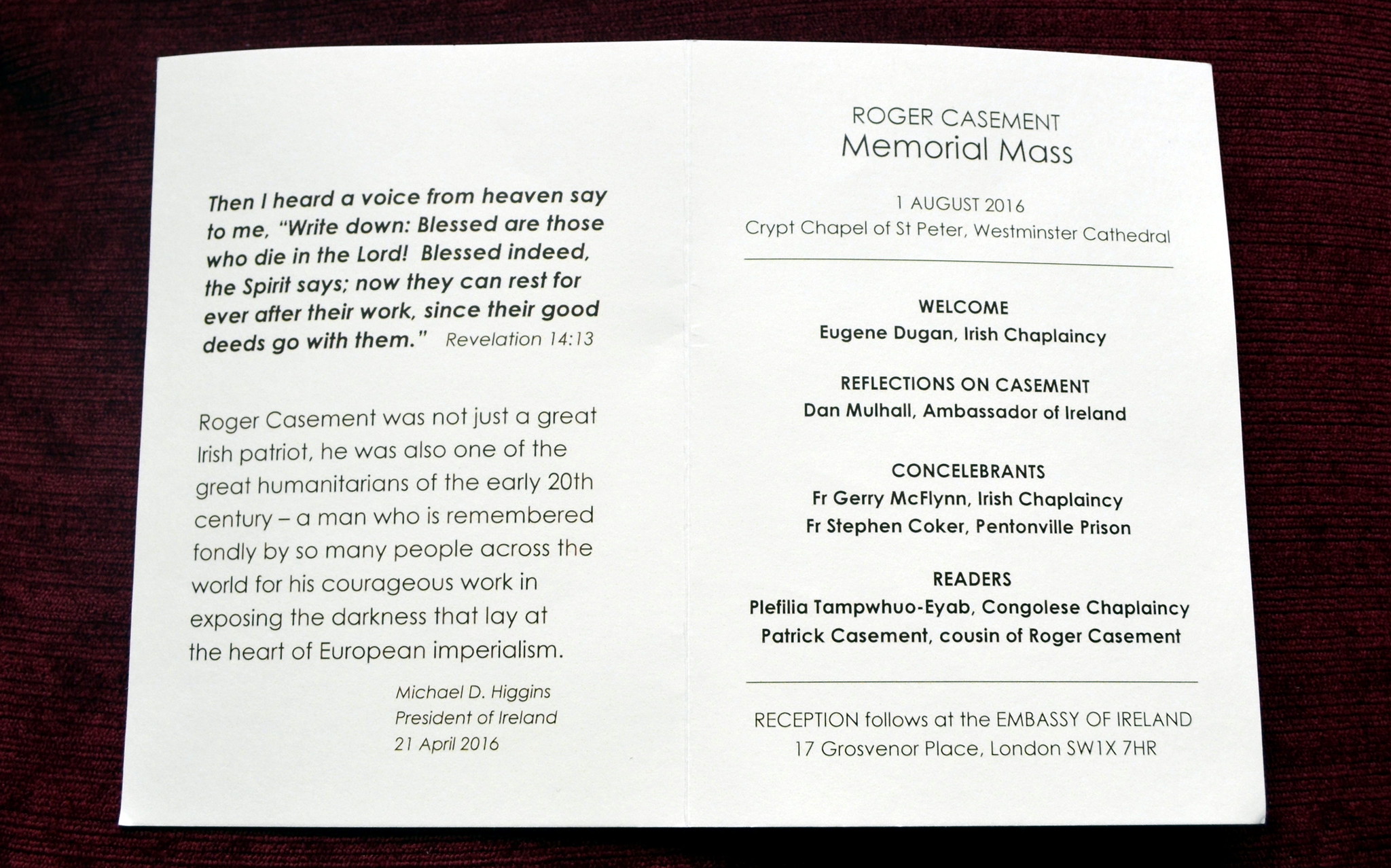The image features a horizontal white card, set against a burgundy surface. On the left side of the card, in black print, there's a paragraph that reads, "Then I heard a voice from heaven say to me, write down, 'Blessed are those who die in the Lord, blessed indeed,' the spirit says. 'Now they can rest forever after their work since their good deeds go with them.'" This text is from Revelation 14:13. Beneath it, another paragraph states, "Roger Casement was not just a great Irish patriot; he was one of the great humanitarians of the early 20th century, a man who is remembered fondly by so many people across the world for his courageous work in exposing the darkness that lay at the heart of European imperialism." This quote is attributed to Michael D. Higgins, President of Ireland, dated 21st April 2016.

On the right side of the card, another section in non-bold print reads "Roger Casement Memorial Mass," dated "1st August 2014." Below this, there are underlined subsections titled "Welcome," "Reflections on Casements," "Consilbrance," "Readers," and details regarding the reception location. At the bottom, another non-bold paragraph appears, providing further details about the event. The entire layout is meticulous, with specific parts of the text emphasized through the use of bold and underlined fonts.